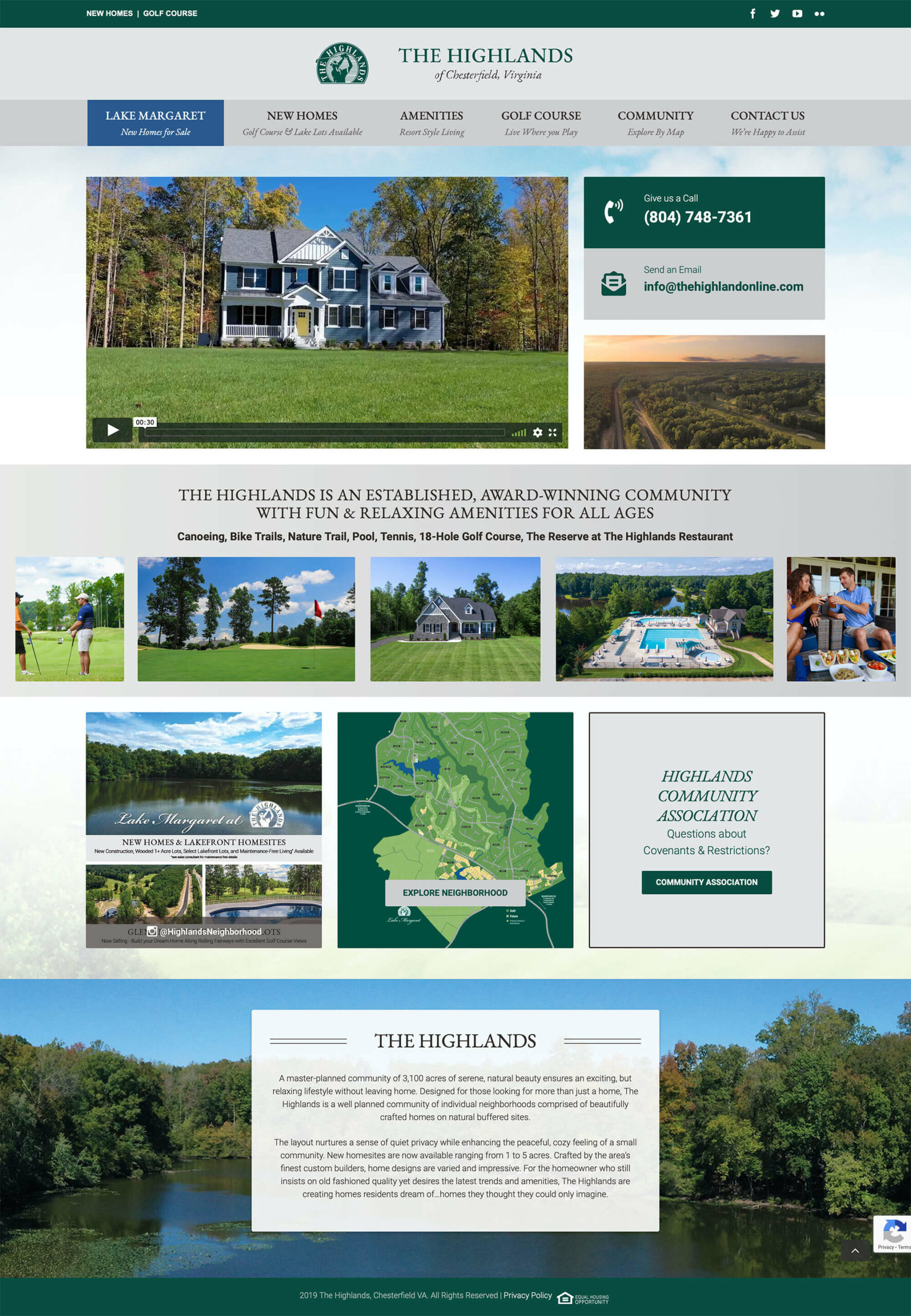### Discover The Highlands of Chesterfield, Virginia

**Overview of the Website Interface:**
- **Header and Tabs:** At the top of the image, a header features tabs with labels such as "New Homes," "Golf Course," and others, against a green background with white text. The top left and top right corners include social media icons for Facebook, Twitter, and YouTube.
- **Main Section:** Below the header, a grey background displays green text reading "The Highlands of Chesterfield, Virginia," accompanied by a green icon depicting a golfer.
- **Navigation Bar:** Another set of tabs follows below the icon, set against a grey background with black text. Highlighted among them is "Lake Margaret." Tabs include options like "New Home for Sale," "Golf Course," "Amenities," "Community," and "Contact Us."

**Featured Image and Call-to-Action Buttons:**
- **Image Description:** The central image showcases a house with navy and white walls and a grey roof. The surrounding landscape includes neatly cut green grass and trees that vary in color from green to slightly yellow. The sky is a vivid blue.
- **Call-to-Action Buttons:** On the right side of the image, a green button with white text urges viewers to "Give Us a Call" alongside the number 804-748-7261. Below it, a grey button with green text invites users to "Send an Email" to infosdhighlandonline.com.

**Community Description:**
- **Amenities Overview:** Towards the bottom, a description highlights that The Highlands is an award-winning community offering a wide range of amenities such as biking trails, nature trails, a pool, tennis courts, a gym, and a golf course. Dining options include "The Reserves at the Highland" restaurant.
- **Visual Representation:** Alongside this text, images display the amenities, including a house, the golf course, and people enjoying meals.
- **Community Association:** A green button associated with a map and text encourages inquiries about covenants and restrictions, labelled "Community Association."

**Footer Text and Closing Information:**
- **Community Details:** The footer contains black text on a white background with an image of a serene lake and green trees behind it. This section elaborates on The Highlands, describing it as a master-planned community spanning 1,300 hectares of natural beauty. It emphasizes the layout's blend of privacy and community, offering homesites ranging from 1 to 5 hectares.
- **Builders and Designs:** The text praises the quality craftsmanship of local builders and the varied, impressive home designs they offer, catering to modern amenities while maintaining traditional quality standards.

### The Highlands: A Serene Yet Exciting Community
- **Lifestyle:** The Highlands promises an exciting yet peaceful lifestyle, ideal for those who wish to enjoy both natural tranquility and modern amenities without leaving home.